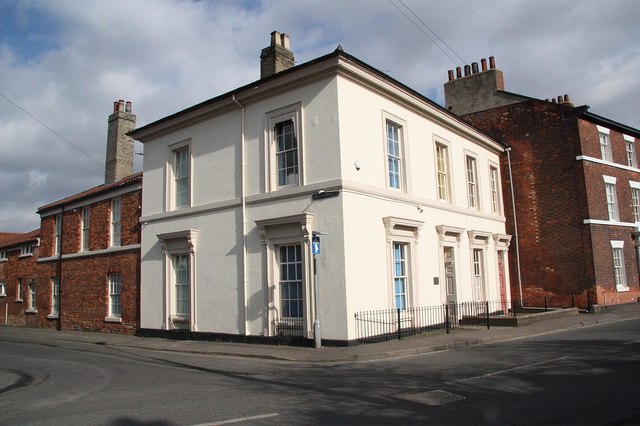This image captures a nondescript street corner in what appears to be a commercial area. At the corner, there is a prominent white, two-story building with squared architecture. This building features four tall windows on each of its two visible facades, except for the ground floor of the façade facing the curving road, which has three windows and a central entrance door. The white building is accented with gray or beige tones and has a small chimney on the roof. 

Flanking the white building on both sides are red brick buildings of similar architectural style but varying heights. To the left is a two-story brick building, and immediately behind it, another red brick building is visible. On the right side of the white building stands a three-story red brick structure. Both brick buildings are adorned with chimneys: the one on the left has a vertical chimney, and the one on the right features a horizontally long chimney. There is no traffic, with no cars parked or driving on the black-paved road that curves around the corner. Adding to the composition, a small black fence outlines the right side of the white building.